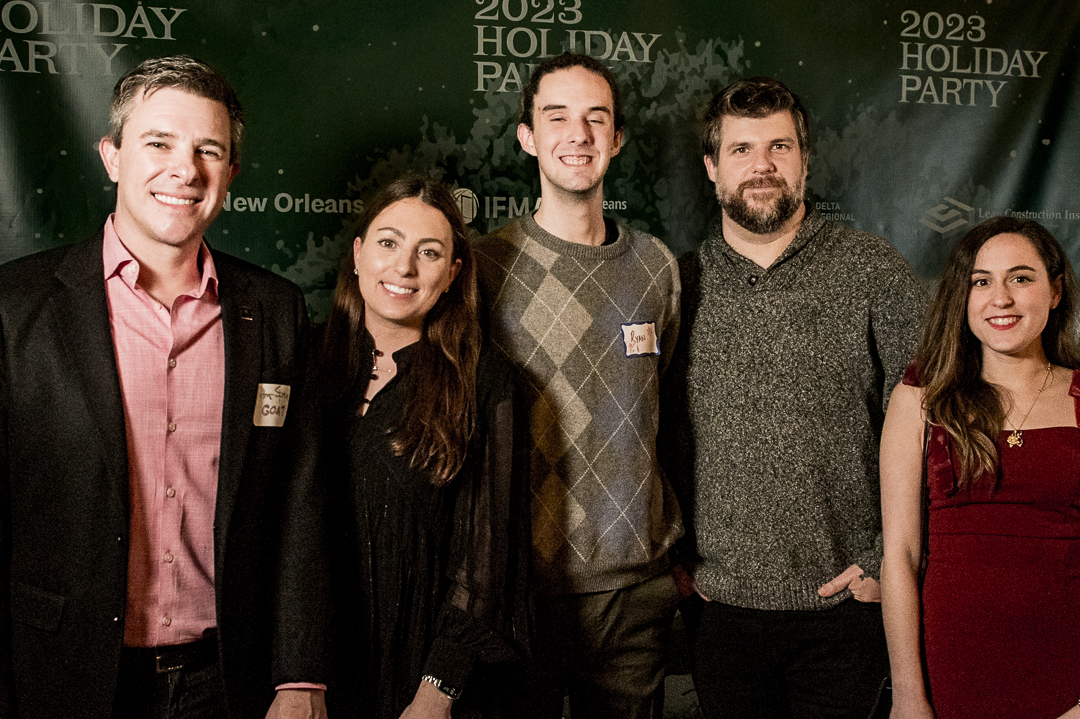The image captures five individuals posing in front of a banner that reads "2023 Holiday Party" and features additional text, including "New Orleans IFM" and an advertisement for a construction company. The setting resembles a red carpet event. 

From left to right:

1. A man with brownish-gray hair, wearing a salmon-colored, long-sleeved, collared button-down shirt paired with a black suit jacket. He is smiling and displaying a name tag.
2. A woman with shoulder-length, long brown hair, adorned with earrings, smiling and dressed in a black blouse with sheer long sleeves.
3. A man dressed in a khaki-toned argyle sweater, described as skinny and wiry, also smiling.
4. An older man with a mustache and short beard, wearing a heavy, speckled sweater in khaki tones.
5. A young woman with long brown hair, wearing a sleeveless burgundy evening dress.

The group appears to be in their mid to late 20s, except for the older man, and the two women look like they might be related.